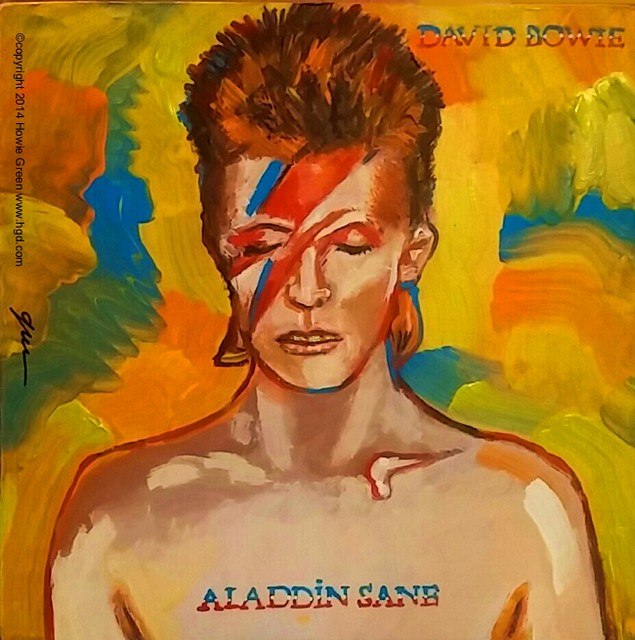The image depicts a vibrant painting of David Bowie, specifically capturing his iconic look from the "Aladdin Sane" album cover. Bowie is the central focus, shown from the chest up with his eyes closed and looking downward. His hair is styled in the distinctive spiky red hairdo synonymous with his Ziggy Stardust persona, and he bears the red and blue lightning bolt across his face. The painting is brightly colored, with a background featuring dynamic and mixed hues of yellow, orange, blue, and green, reminiscent of the Fauve movement. The skin tones of Bowie are rendered in rich, orangey-brown shades, with pronounced features due to the painting style.

Additional details include the words "Aladdin Sane" prominently displayed on his chest, making the album's identity unmistakable. In the top right corner, the name "David Bowie" is clearly visible. The top left corner holds the copyright information, dated 2014, along with the artist's name, website, and a signature. The artwork’s vivid colors and painterly style offer a unique, artistic interpretation of the classic album cover.